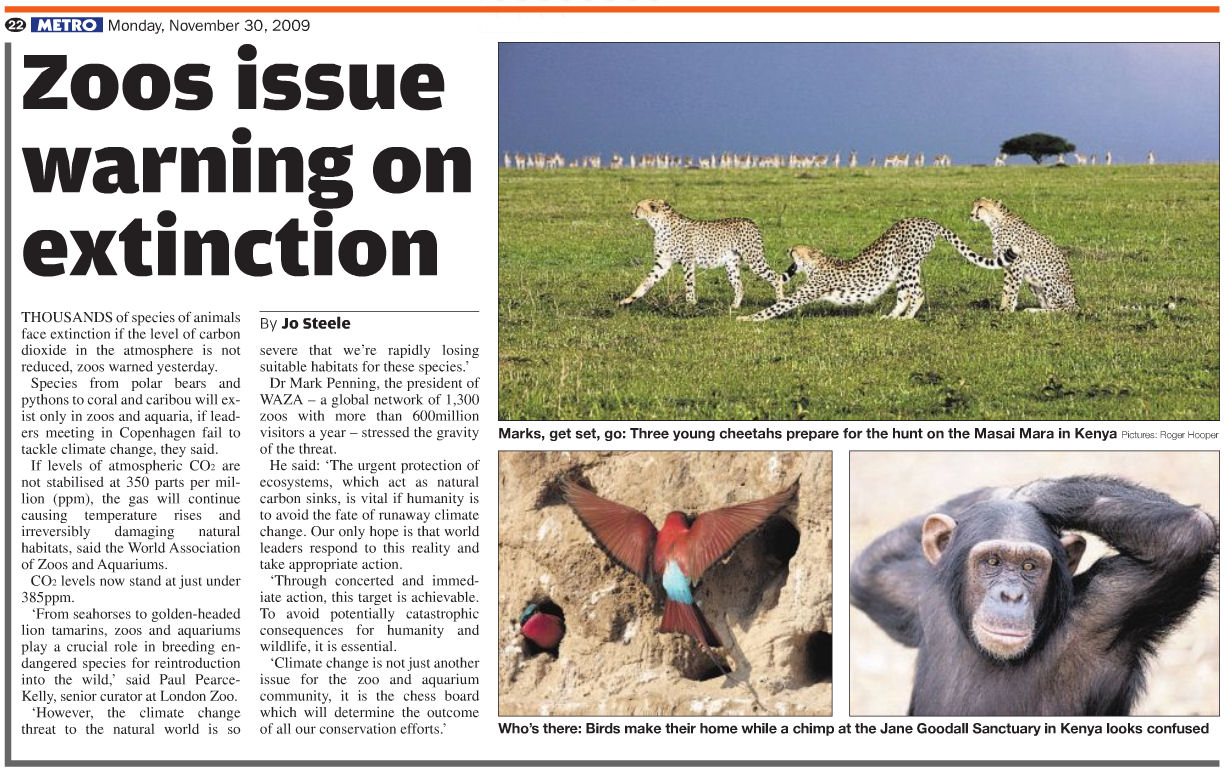**Detailed Caption:**

A newspaper article from Metro, dated Monday, November 30th, 2009, features in the upper right-hand corner, white lettering on a blue background. The headline "Zoos Issue Warning on Extinction" is prominently displayed in large black letters. Below this headline is a photograph depicting three cheetahs: one walking, one stretching, and one sitting. The background showcases a dimly lit savannah landscape with a solitary tree and a miscible sky that appears dark and stormy. The caption for this image reads, "Ready, Set, Go: Three young cheetahs prepare for the hunt on the Maasai Mara in Kenya."

Beneath the cheetah photograph, there's an image of vibrant red birds, with a particular focus on one bird perched on a rock with its wings extended. This image is captioned, "Who's There: Birds make their home while a chimp at the Jane Goodall Sanctuary in Kenya looks confused." 

Next to the birds, an image of a chimpanzee at the Jane Goodall Sanctuary is displayed. The chimpanzee is shown with an inquisitive expression, hands raised, looking to the side with a serious demeanor.

The accompanying article, authored by Joe Steele, elaborates on the urgent warning issued by zoos, highlighting that thousands of animal species face extinction if carbon dioxide levels in the atmosphere are not significantly reduced. The layout of the article is framed with a red bar at the top and a black border outlining the left side and bottom.